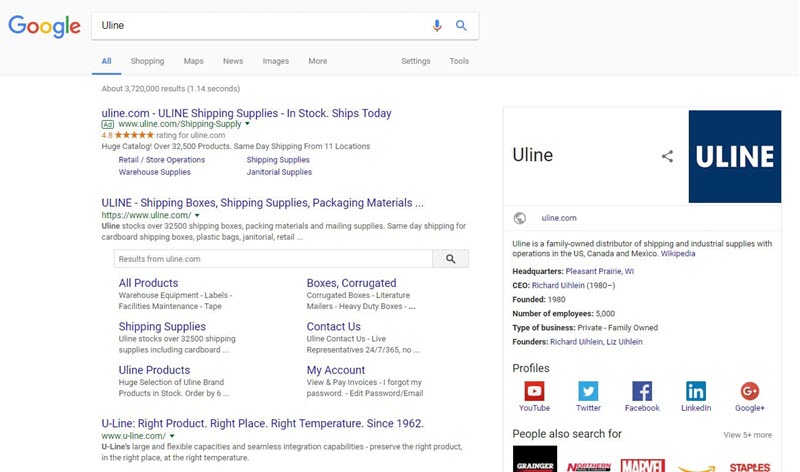A Google search results page is displayed, showcasing a search query for "ULINE." In the top-left corner, the Google logo is prominently shown in its iconic colors: blue, red, yellow, and green. The search bar contains the term "ULINE," and just below it, the navigation options: "All," "Shopping," "Maps," "News," "Images," "More," "Settings," and "Tools" are listed. The "All" option is highlighted in blue, indicating it is selected, while the others remain in gray.

The results page indicates approximately 3,720,000 results were found in 1.14 seconds. The first search result is an advertisement for Uline, a well-known supplier of shipping supplies. The ad summary states: "Uline.com – Uline Shipping Supplies in Stock. Ships Today." The advertisement also mentions Uline's 4.8-star rating and highlights its vast inventory of over 32,500 products available for same-day shipping from 11 locations. Product categories include retail/store operations, warehouse supplies, shipping supplies, and janitorial supplies.

The actual search result beneath the ad further describes Uline's extensive inventory, emphasizing shipping boxes, packaging materials, and mailing supplies. This result reiterates Uline's commitment to same-day shipping for a wide array of items, such as cardboard shipping boxes, plastic bags, janitorial supplies, and more. Additional links are displayed for detailed categories like "All Products," "Shipping Supplies," "Uline Products," "Boxes," "Corrugated," as well as options for contacting Uline and accessing personal accounts.